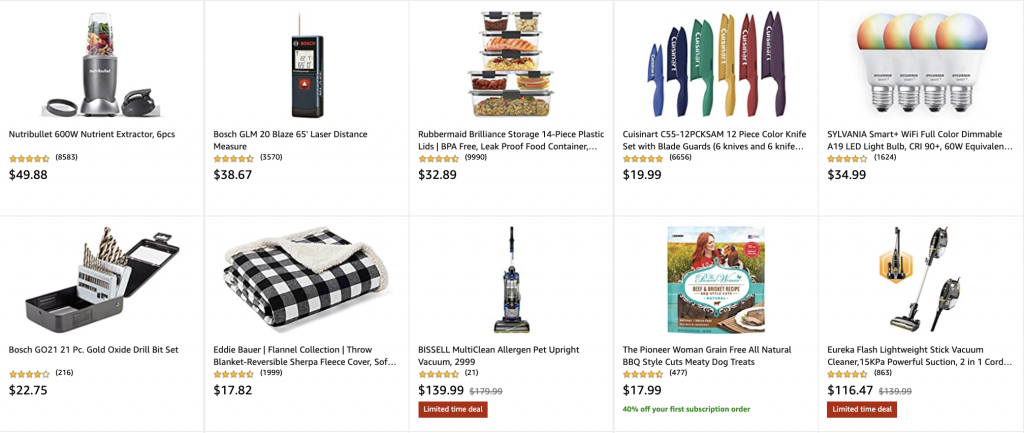This webpage from an e-commerce site resembles Amazon, featuring a selection of items for sale in a grid layout. The page displays 10 products, with 5 items presented across the top row and 5 across the bottom. Each product is showcased within its own square section.

**Top Row:**
1. **Nutribullet 600 Watt Nutrient Extractor (6-piece)** - $49.88
2. **Bosch GLM 20 Blaze 65-Foot Laser Distance Measure** - $38.67
3. **Rubbermaid Brilliance Storage Set (14-piece with Plastic Lids)** - $32.89
4. **Cuisinart C55-12PCKSAM 12-Piece Color Knife Set** - $19.99
5. **Sylvania Smart+ WiFi Color Dimmable A19 LED Light Bulb** - $34.99

**Bottom Row:**
1. **Set of Drill Bits** - $22.75
2. **Eddie Bauer Flannel Throw Blanket** - $17.82
3. **Bissell Multi-Clean Pet Upright Vacuum** - $139.99
4. **The Pioneer Woman Grain-Free All-Natural BBQ Style Cuts Dog Treats** - $17.99
5. **Eureka Glass Lightweight Stick Vacuum Cleaner** - $116.47

Each item is clearly separated and easily identifiable, allowing users to quickly browse through a variety of tools, household items, and pet care products.